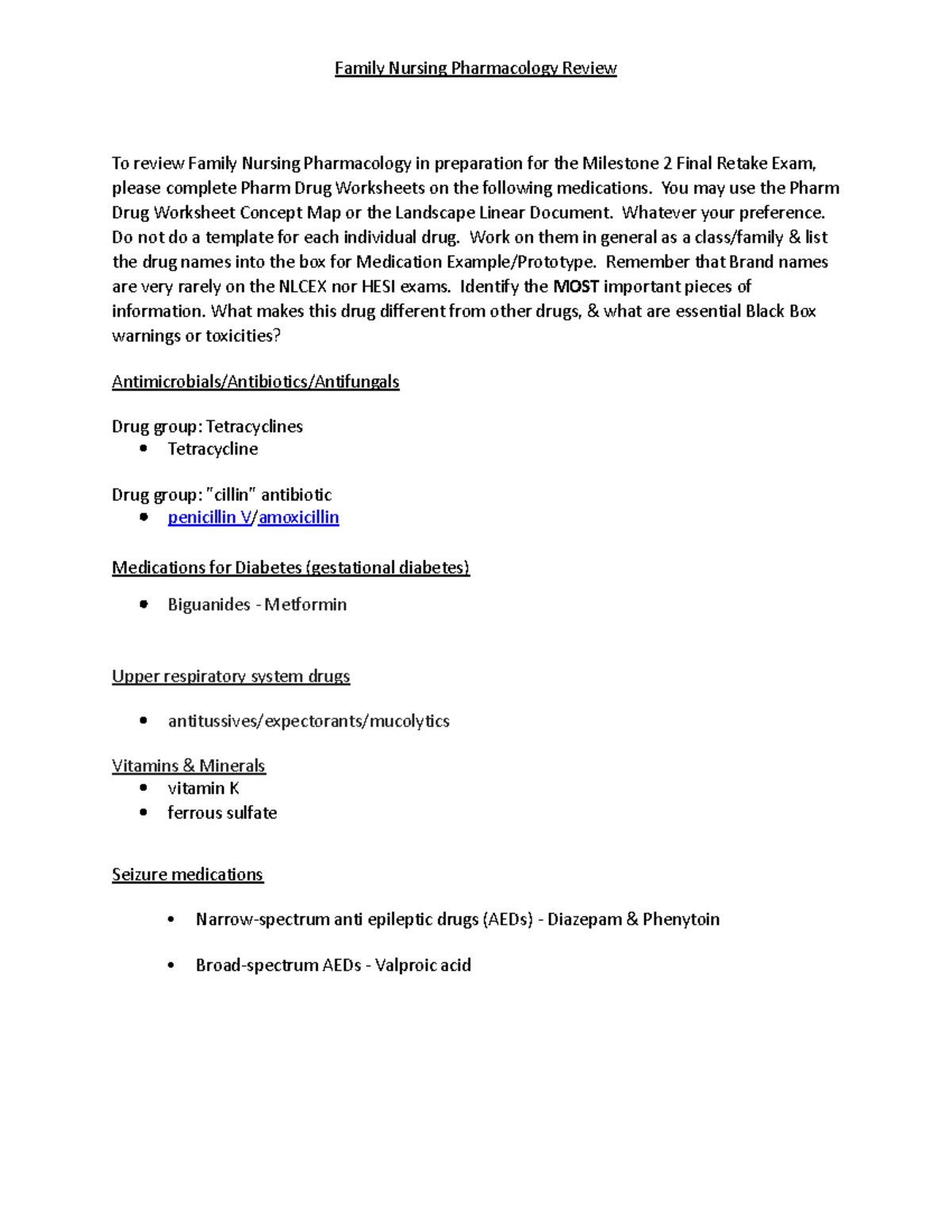The image is a screenshot featuring text on a white background, with the text in black. At the very top, there is a heading: "Family Nursing Pharmacology Review," which is underlined in black for emphasis. Below the heading, there is a detailed instruction: 

"To review Family Nursing Pharmacology in preparation for the Milestone 2 Final Retake Exam, please complete Pharm Drug Worksheets on the following medications. You may use the Pharm Drug Worksheet Concept Map or the Landscape Linear Document based on your preference. Do not create a template for each individual drug. Instead, work on them generally as a class or family and list the drug names in the 'medication example/prototype' box. Remember that brand names are very rarely included in the NCLEX or HESI exams. Identify the MOST important pieces of information – note that 'MOST' is capitalized and bolded for emphasis. Focus on what makes each drug different from others and any essential black box warnings or toxicities."

Below this paragraph, there is another section titled "Antimicrobials, Antibiotics, Antifungals," which is also underlined in black. The text continues with "Drug Group: Tetracyclines, Tetracycline," indicating the specific class of drugs for which the worksheet should be completed.